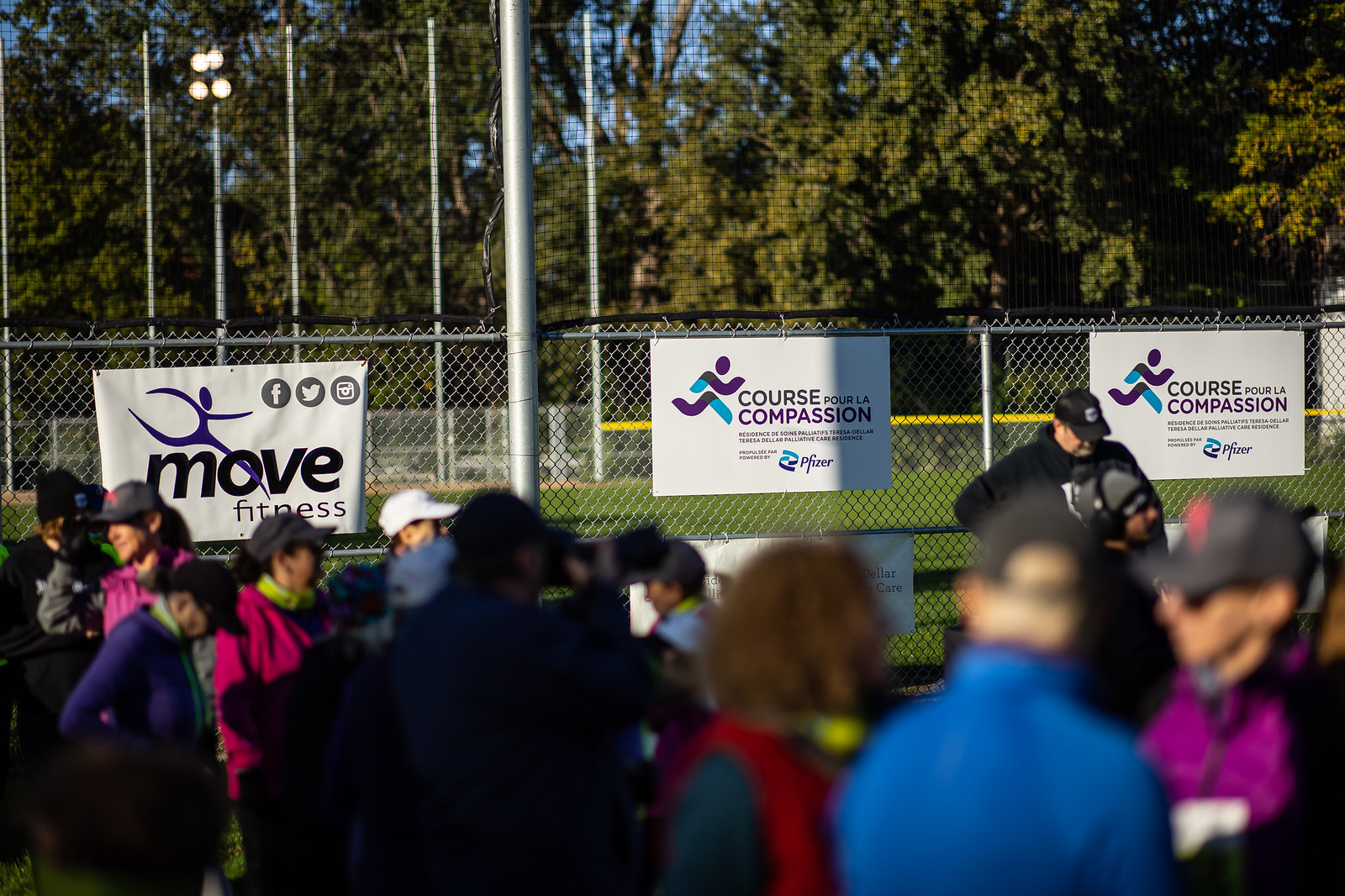This is a detailed photograph of an outdoor sporting event set in a park. The image is horizontal and rectangular, capturing the scene from behind a group of people, mostly mature adults, dressed in various colored athletic jackets and baseball caps, indicating it might be a chilly but sunny day. The photo seems to depict a community-based event, possibly a walking or athletic activity preparing to start. In the foreground, the people are standing near a chain-link fence adorned with several white banners. Clear promotional messages are visible, including ones that say "Move Fitness" and "Course For Love Compassion By Pfizer." Beyond the fence, the setting transitions into a lightly visible tennis court with a net stretched across the middle, indicating it's an outdoor sports ground. The court features several light poles, suggesting it is used during evenings as well. The backdrop consists of a dense line of trees with a narrow gap revealing a touch of blue sky. No players are present on the tennis court, reaffirming that the focus is on the gathering of people in the foreground. The setting exudes a communal and local atmosphere rather than that of a professional sports venue.